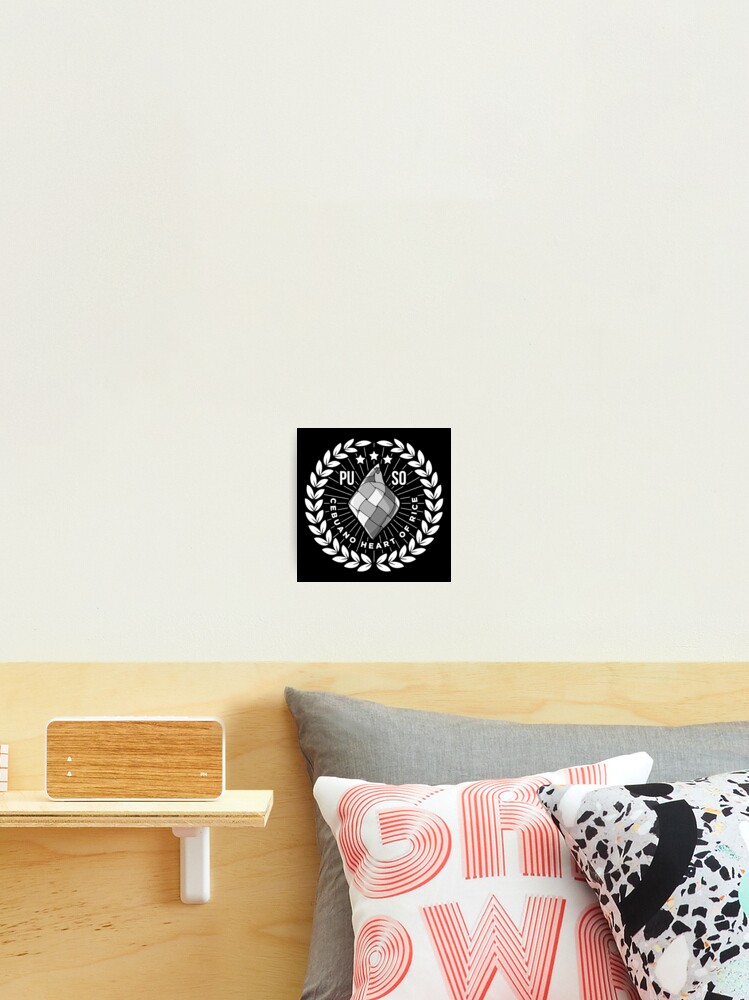The image showcases a tastefully decorated bedroom with a harmonious blend of modern and rustic elements. Dominating the upper portion of the scene is a white wall adorned with a rectangular emblem featuring the initials "PUSO" and the phrase "Sibuano Heart of Rice." Surrounding this text is a circular design, possibly depicting stylized rice grains before harvest, adding a cultural touch to the decor. Below this, a blond wood headboard spans the width, providing a warm contrast.

In the foreground, a series of pillows add texture and color to the arrangement. The first pillow exhibits a black and white print, while the second pillow beneath it is white with bold orange letters, including a visible "G," "R," and "W." Behind these, a solid gray pillow anchors the trio against the headboard.

To the left, a sleek, modern shelf made of plain plywood and supported by white braces hosts a futuristic-looking device. This device, possibly a radio, sports a minimalist plywood front devoid of visible dials, enhancing the room's contemporary aesthetic. The overall setup, while seemingly eclectic, creates a cohesive and visually engaging display.